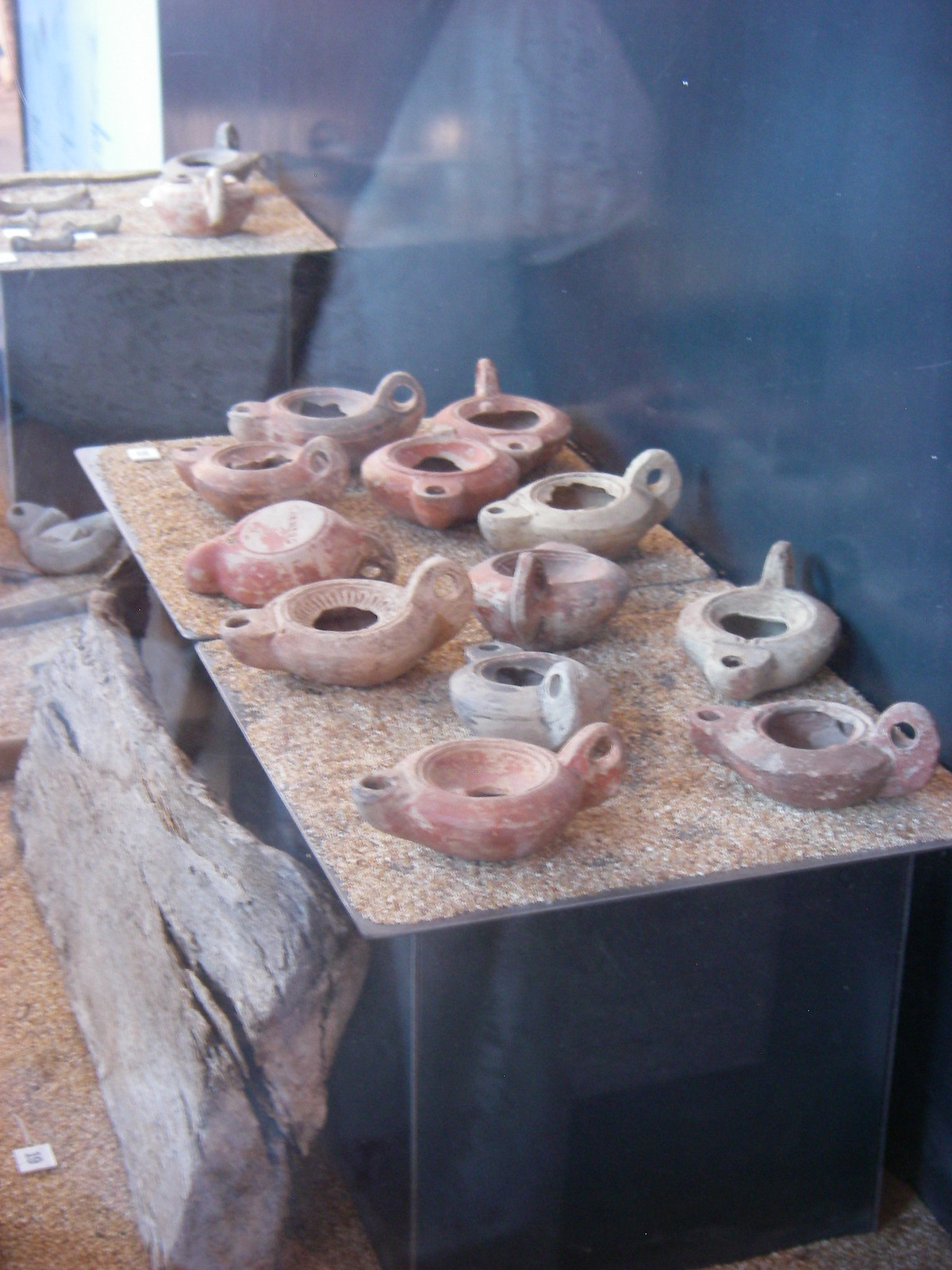The color photograph, taken in a portrait orientation, showcases a museum display viewed through a pane of glass, evidenced by the soft reflections in the foreground. In the top-left corner, there seems to be an arm with a white sleeve, possibly belonging to the photographer. The display consists of ancient ceramic pottery, characterized by their distinctive spouts and handles, resembling gravy boats or genie bottles. These ceramics, in various hues from darker browns and brick red to light sandy browns and grayish off-whites, are arranged on tables. One of the tables is situated in the foreground against a wall along the right side, while another is positioned in the back left, holding the rest of the pottery. Beside the table on the right, a large piece of a tree trunk leans conspicuously, adding a rustic touch to the display. The floor in the left corner is adorned with what looks like wood chippings, and there are additional, partially obscured items behind the tree trunk, including perhaps another pot and some wooden planks. Notably, one pot is turned upside down on a marble slab, perched on a dark base with split wood leaning against it. Additionally, the number '19' is visible and skewed in the bottom left corner, further indicating its placement in a museum setting.